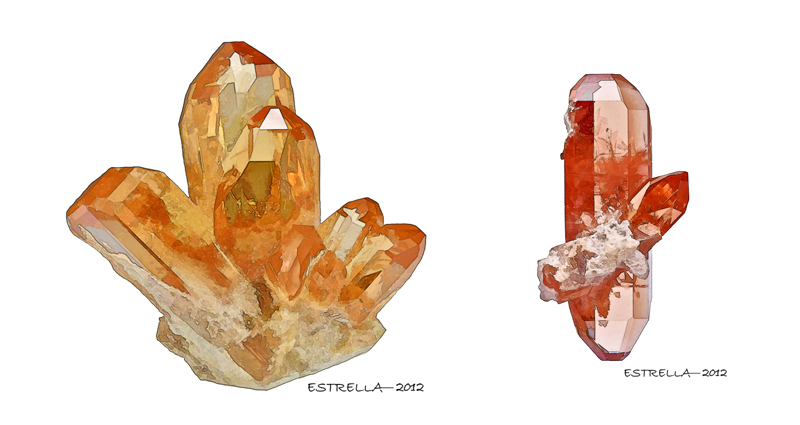This image features artistic depictions of two crystals against a white background. On the left side, there is a larger, orange-tinted crystal composed of multiple smaller crystal formations. On the right side, a smaller, red-tinted single crystal is depicted in a cylindrical shape. Both crystals have been rendered with highlights and shadows, giving them a shiny, semi-transparent appearance. Below each crystal, the inscription "Estrella 2012" is subtly placed in a small font. The overall style of the image is more illustrative rather than realistic, emphasizing the artistic use of colors and shading.